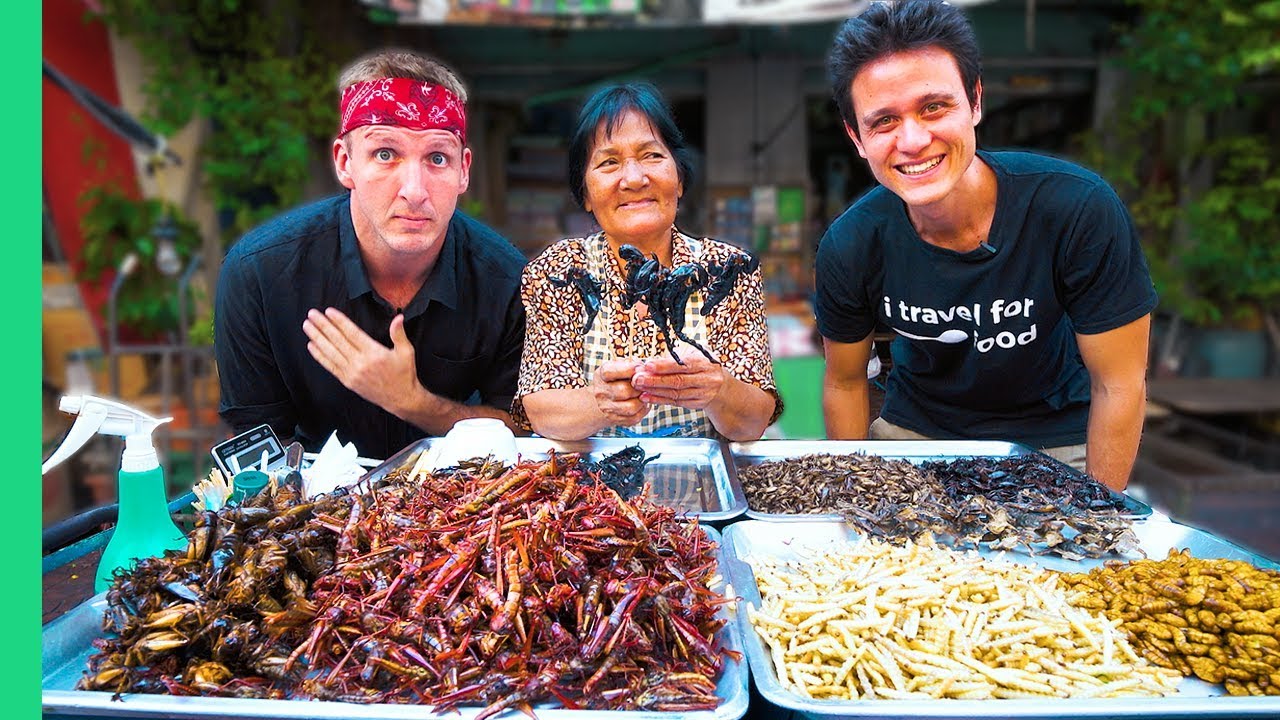In this vibrant and intriguing photograph, three distinctive individuals are captured in front of an impressive display of exotic foods. The two men flank a woman, all facing the camera with an air of camaraderie. To the left, a Caucasian man with light hair and striking blue eyes stands confidently, sporting a red bandana and an unbuttoned black collared shirt. On the right, a South Asian man wears a black T-shirt emblazoned with the phrase "I travel for food" along with an image of a spoon, and has a microphone clipped to his shirt, hinting at his role as a food YouTuber.

In the center stands a dark-skinned woman with dark hair, possibly South Asian, dressed in a floral blouse in shades of tan, brown, and white, complemented by an apron. She holds a skewer of scorpions, adding to the adventurous spirit of the scene. In front of them, a variety of critters are spread across several tin trays, piled high with mealworms, centipedes, and other insects, showcasing a unique array of delicacies. A spray bottle and a scale can also be seen among the trays, emphasizing the meticulous setup of this food presentation. The setting suggests an exploration of global culinary practices, likely for a blog or YouTube channel.